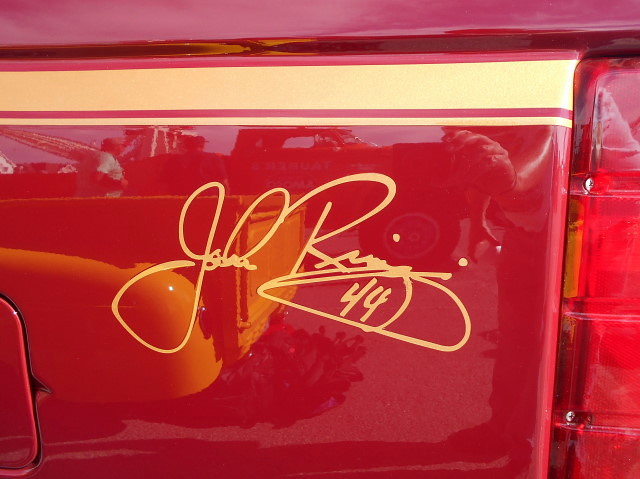This detailed image showcases the rear fender of a bright fire-engine-red car, adorned with a gold pinstripe. Prominently featured on the fender is a signature in elaborate gold cursive script, reading "John Riggins," with the number 44 intricately embedded within the last name. The right side of the frame captures the red taillight, with two gold stripes extending from it—a thicker one on top and a thinner one below. Just left of the gas cap, the door of the gas tube is visible. The car's glossy, reflective surface reveals the image of a yellow pickup truck, hinting at the scene surrounding the vehicle. Additionally, the reflection includes details such as a large truck in the background, a person capturing the photo on their phone, and other nearby individuals.